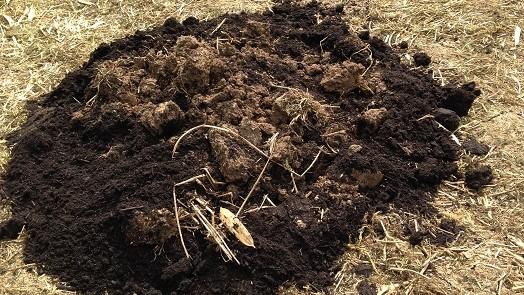In this detailed photograph taken inside a barn on a farm, we see a large, dark brown pile of manure, which forms a nearly spherical mound with three distinct indents, hinting at it being pressed down by a rake. The manure is mixed with partially chewed or fragmented hay, which stands out in the center with its lighter beige and tan colors. This pile lies on a flat surface of dry hay that serves as the background. The surrounding hay is uniformly beige and tan, contrasting with the deep, rich brown of the manure. The image is horizontal, and the clarity of the details suggests this is a real-life scene, possibly evocative of a spot where manure has been collected and mixed with hay, rather than a large hole dug in the ground.